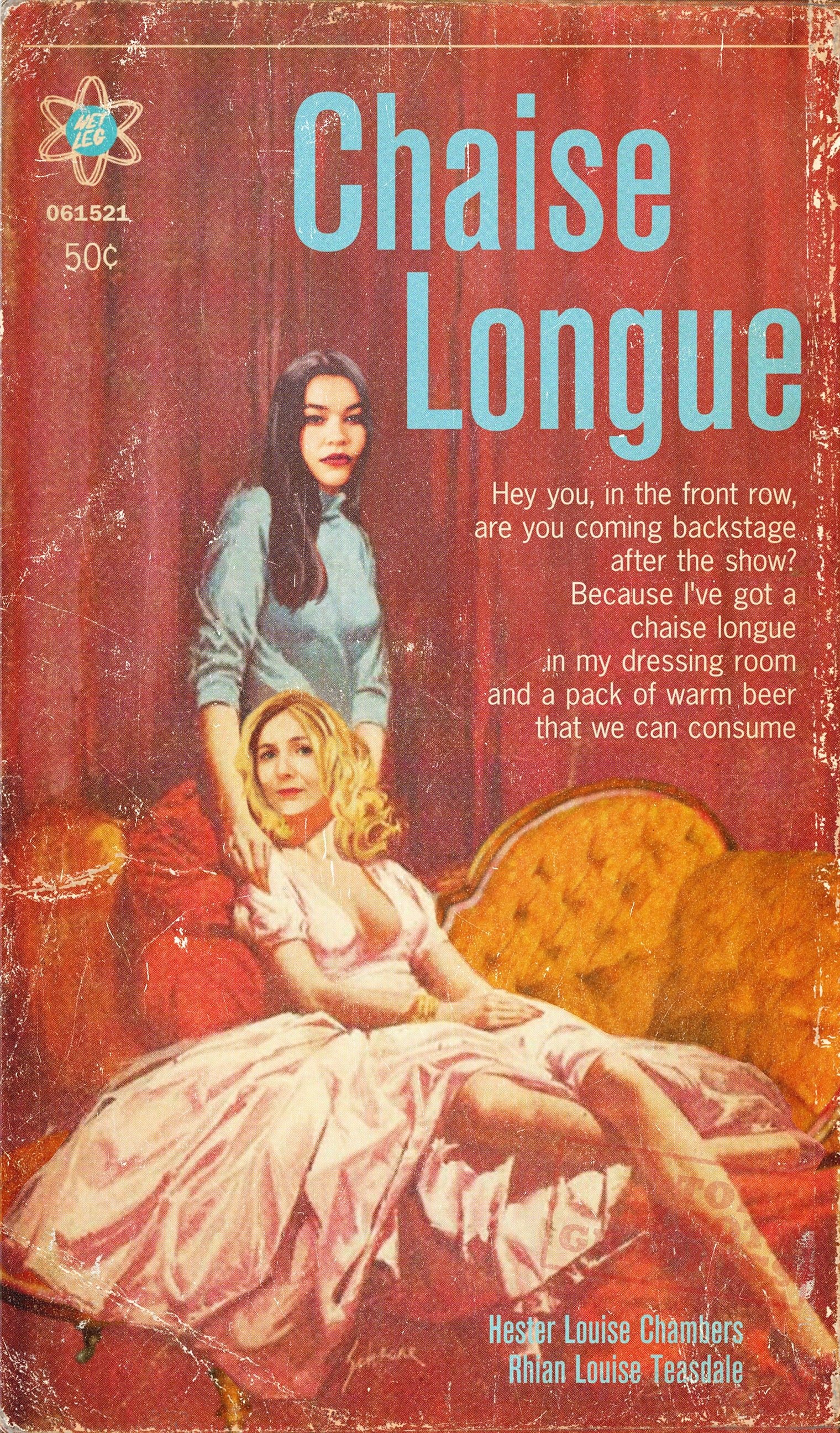The image depicts a vintage magazine or playbook cover with a rich red curtain backdrop. Dominating the center is a yellow chaise lounge on which sits a blonde woman wearing a pink, low-cut, full dress that reveals her legs from the knee down. Behind her stands another woman with dark hair, dressed in a blue turtleneck top with three-quarter sleeves, resting her hands on the seated woman's shoulders. At the top of the cover, bold blue letters spell out "Chase Lounge" followed by a playful tagline: "Hey, you in the front row, are you coming backstage after the show? Because I've got a Chase Lounge in my dressing room and a pack of warm beer that we can consume." In the upper left corner, there is a star-shaped emblem with the text "NETLAG" (possibly indicating the publisher) alongside the numbers 061521 and a price of 50 cents in cream color. In the bottom right corner, the authors' names, Hester Lewis Chambers and Rhian Lewis Teasdale, are printed in light blue letters. The overall composition suggests an intriguing blend of retro charm and theatrical allure.